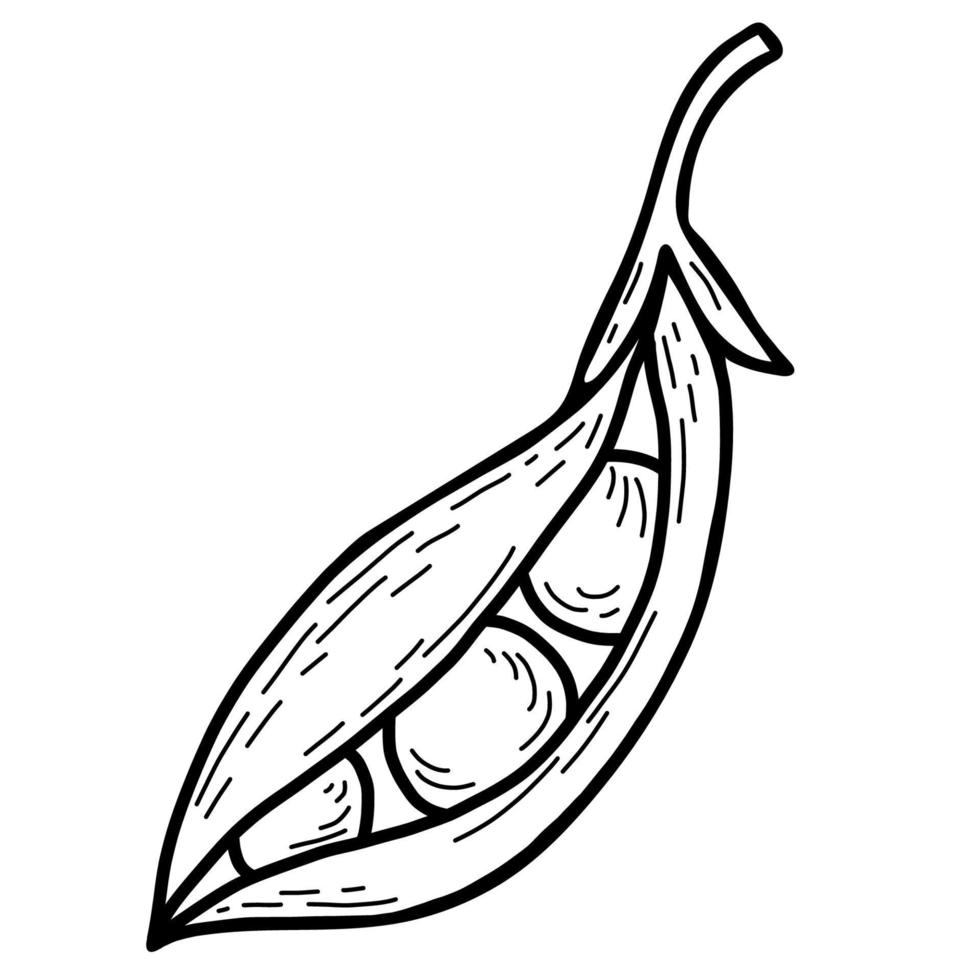This is a detailed black and white illustration, possibly hand-drawn or digitally created, depicting the outline of a pea pod on a stalk. The stalk starts from the top right corner, extending downward before branching into two leaves that curve to the left and right. Below this, the pod narrows at the base and then broadens into an elongated, cat-eye shape. The pod is slightly open at the front, showcasing three peas inside: the largest pea is in the middle, the next largest is towards the top right, and only a small portion of the smallest pea at the bottom is visible. The entire image is enriched with texture lines, including short strokes throughout the stalk, leaves, pod, and peas, adding a dynamic quality to the illustration. The background is plain white, and there is no text within the image.